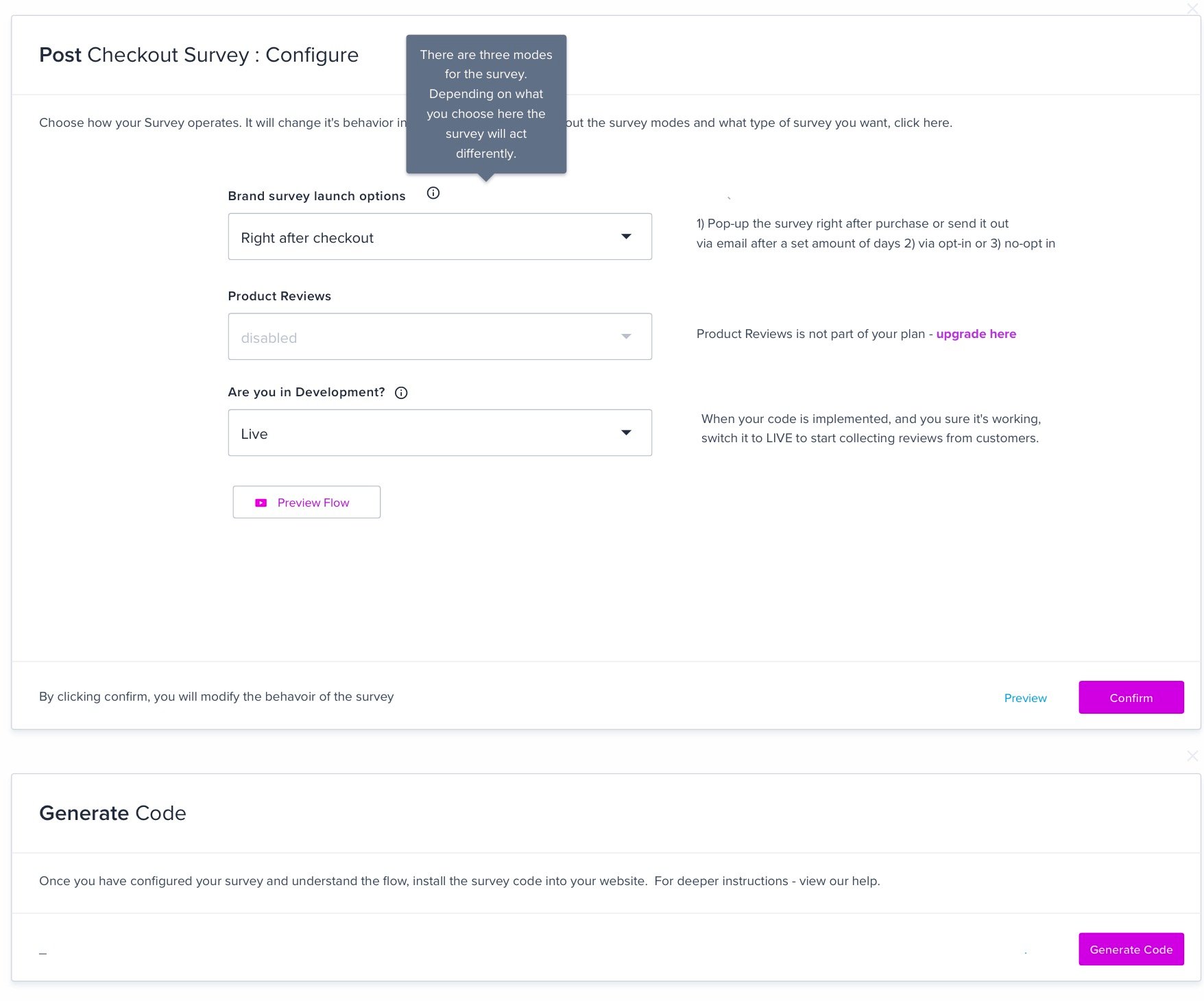Here's a detailed and cleaned-up caption for the described image:

---

The image features a white background with black text positioned at the top, reading "Post Checkout Survey Configured." Below this header, a subheading in black text states, "Choose how the survey operates. It will change behavior." A semi-transparent bluish popup overlays this text, obscuring some content. The visible text following "Behavior" reads, "But a Survey, Survey Models." This section appears to guide the user on selecting the type of survey they want by clicking a designated area.

Within the popup, white text indicates there are "three modules for the survey." It suggests that the survey’s operation varies depending on the module chosen, emphasizing flexibility in survey behavior. Some legibility issues persist but the intent remains clear.

On the left side, black text reads "Brand Serving Launch Options," likely outlining different setup choices for brand-related post-checkout surveys. On the right side of the popup, more black text is present but is difficult to read. However, the phrase "Product Reviews" is identifiable and marked as disabled, along with a note clarifying that "Product Reviews is not part of your plan; you can upgrade it."

Further down, options appear to toggle between "Development" and "Live" states of the survey. Another visible text block, albeit partly illegible, probably refers to managing survey launch conditions.

Below, a clearly visible blue link states "Preview Flow," suggesting an option to review the survey flow before finalizing configurations. Underneath, a square notification reads, "By clicking Confirm, you will modify the behavior of the survey." This indicates a procedural step for finalizing changes either by reviewing or confirming them, highlighted in purple.

Towards the bottom, instructions detail coding steps: "Once you have configured your survey and understand the flow, install the survey code onto your website." For design guidelines, the text suggests consulting their help support. A purple button located in the bottom-right corner of the popup provides further interaction.

---

This comprehensive description covers all visible details and their potential implications in the provided image.